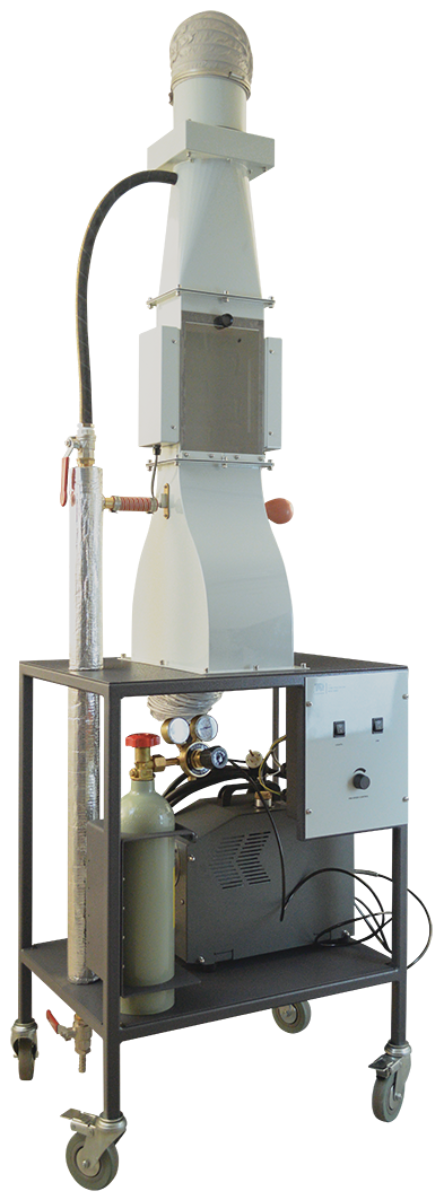The image displays a detailed, colored photograph of a piece of equipment positioned against a plain white background. The focal point is a metal rolling cart with a silverish-brown finish, featuring two shelves supported by four black wheels typical of those found on shopping carts. On the bottom shelf rests a gas cylinder equipped with a red twist knob and a handle, suggesting it contains some type of gas. Adjacent to the cylinder sits a gray or black box with exposed wiring, possibly for controlling the equipment's functions. The top shelf supports a tall, white pillar with some gray accents. A black hose extends from this pillar down to the base, while a prominent red valve nestled at the top of the pillar allows for gas regulation. The apparatus appears to channel the gas up into this upper chamber, hinting at a complex mechanism designed for gas transfer or control.